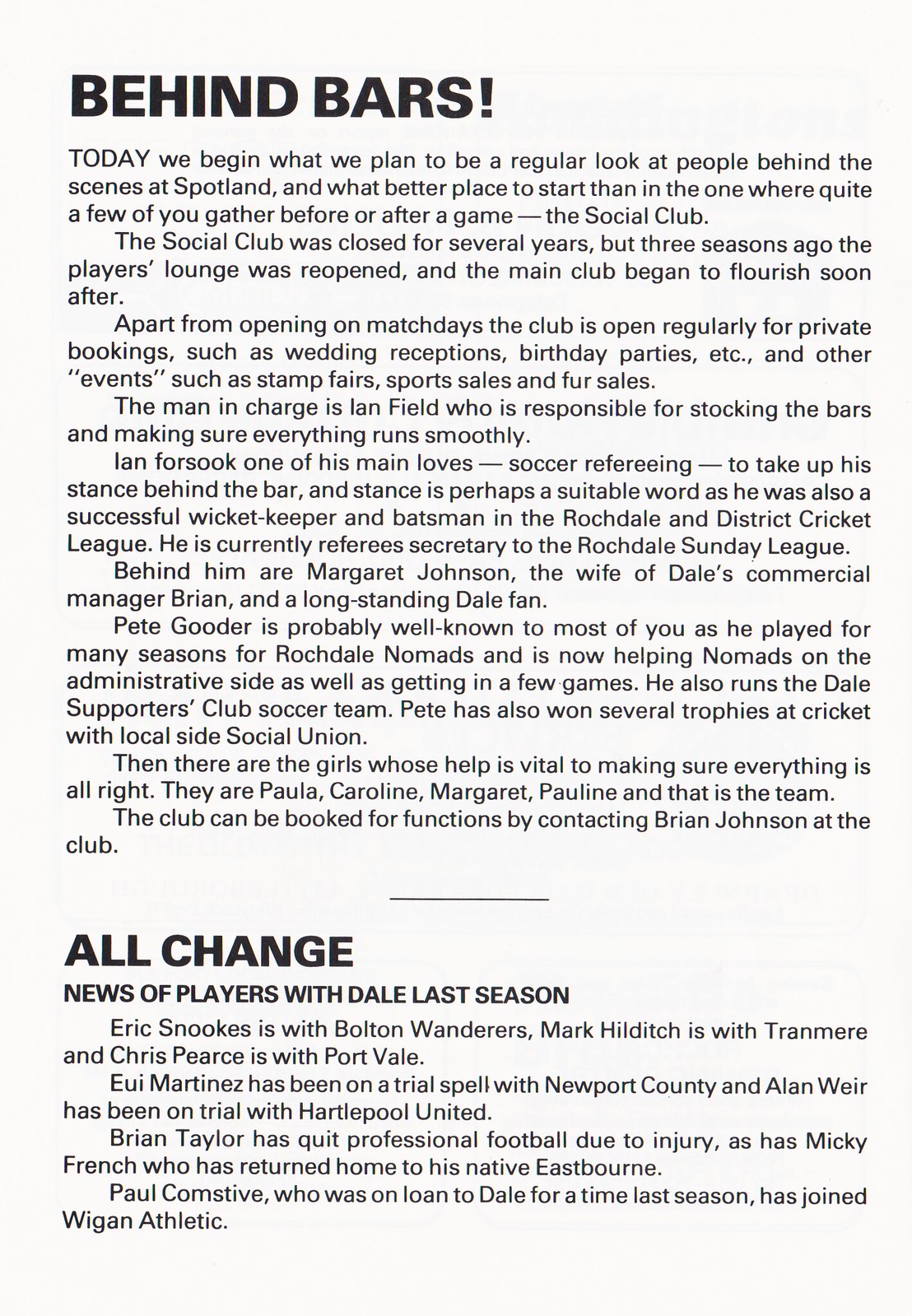This image displays a program insert from a soccer game, featuring an article titled "BEHIND BARS!" on a light gray background with black font. The article begins with the sentence, "Today we begin what we plan to be a regular look at people behind the scenes at Spotland, and what better place to start than in the one where quite a few of you gather before or after a game: the social club." The social club's history is detailed, noting its closure for several years and subsequent reopening of the players' lounge three seasons ago, leading to the club's revitalization. It explains that the club now regularly hosts private events such as wedding receptions, birthday parties, stamp fairs, sports sales, and fur sales, in addition to being open on match days. The man overseeing operations is Ian Field, a former soccer referee and current referee secretary for the Rochdale Sunday League, assisted by Margaret Johnson and Pete Goudar, who has a historical connection with the club and its administrative activities. The article highlights that the staff, including Paula, Caroline, Margaret, and Pauline, are essential for the club's smooth operation. Towards the bottom, another section in bold capital letters says "ALL CHANGE," followed by a smaller capitalized subtitle "NEWS OF PLAYERS WITH DALE LAST SEASON," accompanied by several paragraphs of text.